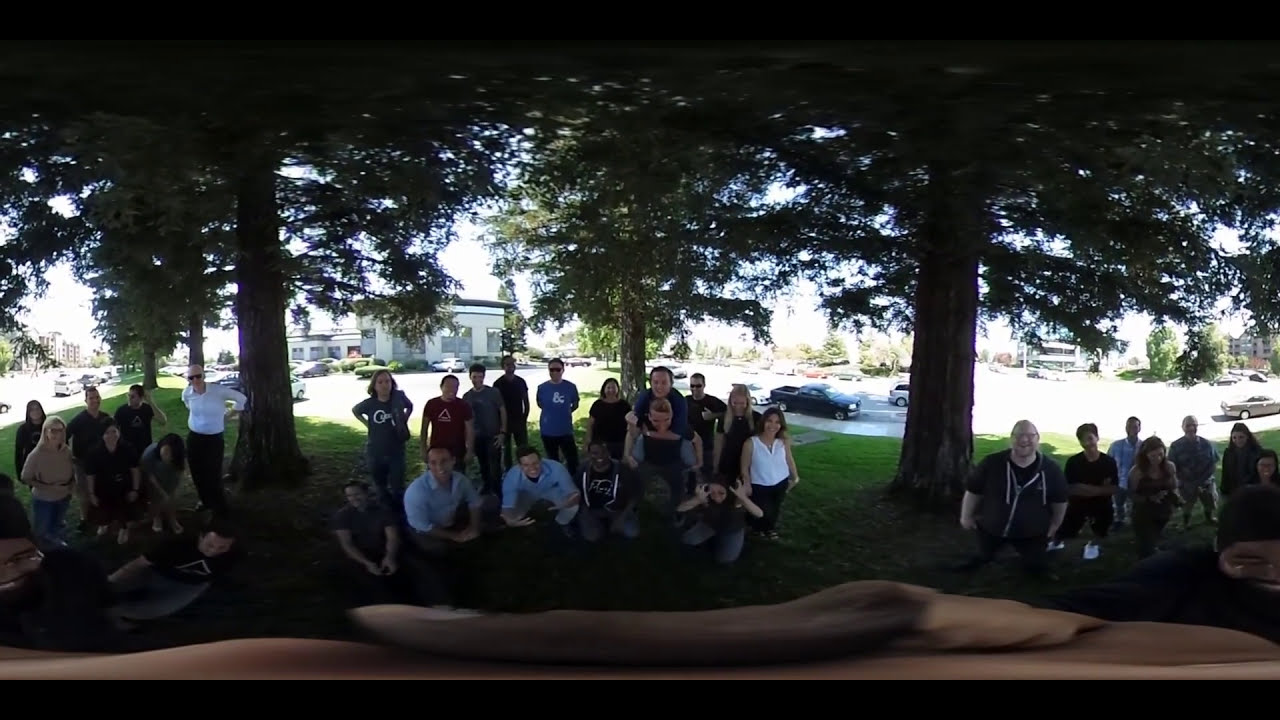The photograph depicts a large outdoor gathering of people in a lush garden, captured with a fisheye filter that gives it a panoramic, wraparound effect. The image is divided into three distinct groups of individuals: one group in the center, another on the left, and the third on the right. Each cluster comprises a mix of people both sitting and standing, with some posing for the camera. Notably, one person in the center group is giving a piggyback ride, adding a playful touch to the scene.

All three groups are positioned under the shade of two large trees with expansive branches and dense foliage, which create dappled shadows on the green grass below. The garden setting is vibrant, with sunlight filtering through the treetops. In the background, a parking lot with about three vehicles is visible, along with a road and distant buildings, which are bathed in more direct sunlight. The image also features a distinctive brown smear along the bottom, possibly an artifact from the panoramic capture process, and black borders at the top and bottom. This gathering, composed predominantly of Caucasians with a few African Americans, suggests a family get-together or similar social event.